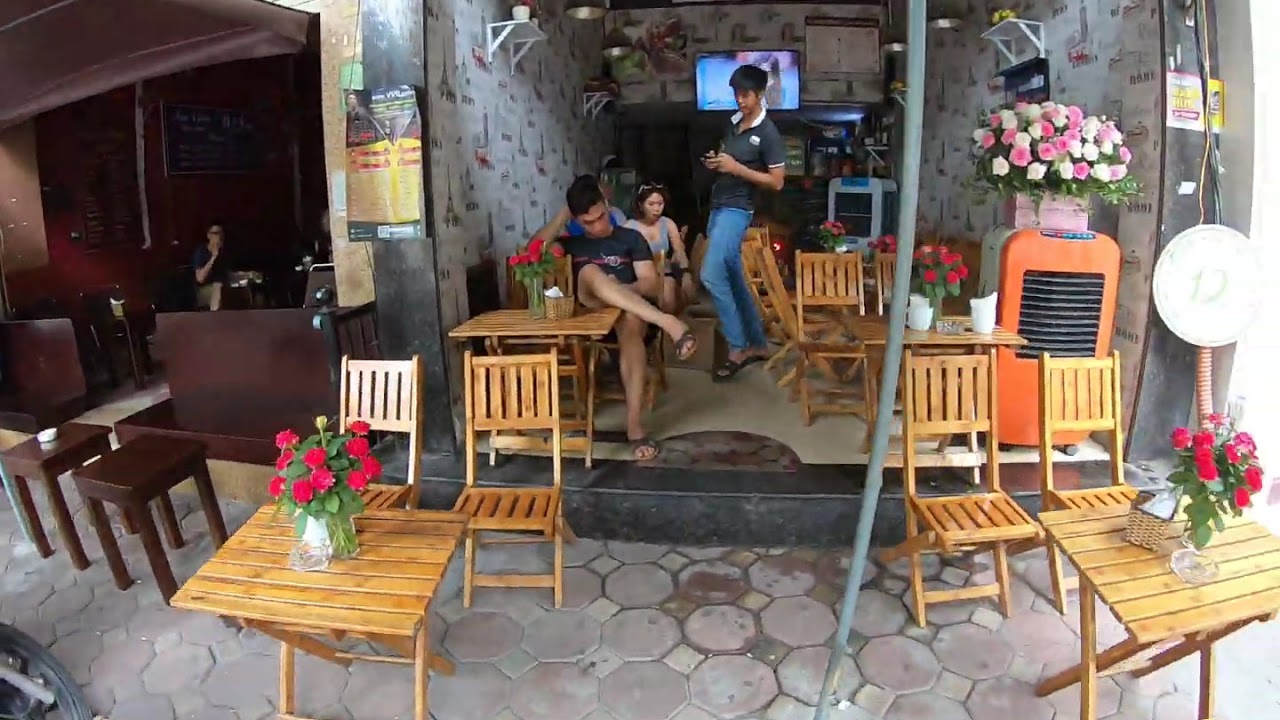This photograph captures a bustling scene of two adjacent storefronts in what appears to be an Asian country, possibly Thailand or the Philippines. The primary focus is a quaint, small café with an open facade composed of light tan, foldable wooden tables and corresponding small wooden chairs set up intermittently. The setting features minimal decoration, save for a TV mounted on the far back wall and vases of red flowers adorning each table, adding a vibrant touch of color. Additionally, a bouquet of pink and white roses sits in a vase toward the right side of the photograph.

In this café, two people are seated at the tables, absorbed in reading or looking at their phones. Between the rows of tables stands an Asian man who appears to be a waiter, dressed casually in jeans, flip-flops, and a green polo shirt with a white collar.

Adjacent to this café is another restaurant characterized by darker wood elements, including dark mahogany wood panels and tables. Despite the contrasting themes, both establishments share a lively atmosphere with patrons either waiting for their orders or enjoying their meals and drinks.